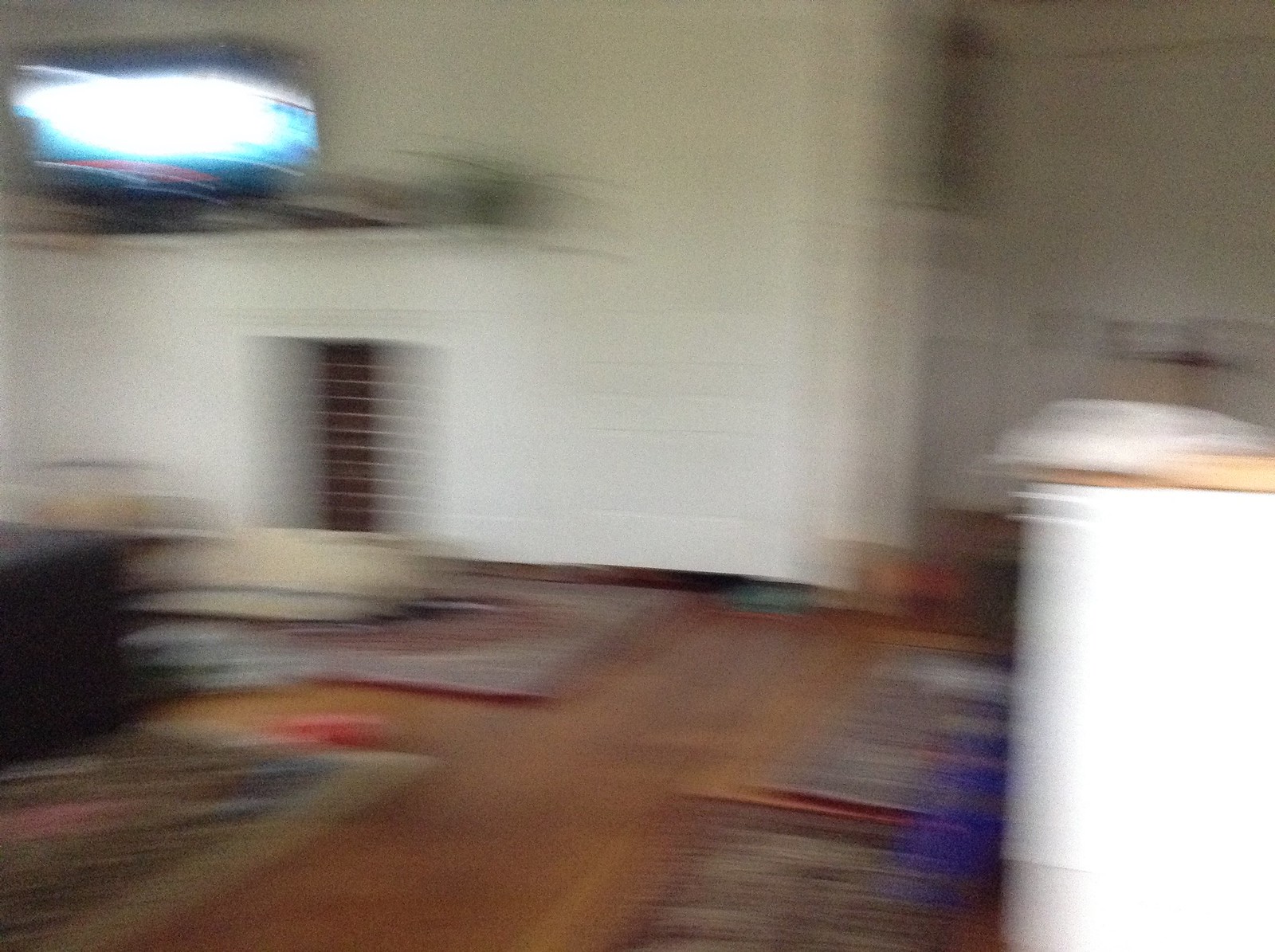This image depicts a very blurry portion of a home living room with several distinguishable features despite the motion blur. The floor is wooden and covered with four different area rugs. On the left, there is a large area rug with a rectangular wooden coffee table on top. A black cube-like piece of furniture is also visible in this section. To the right, two small area rugs are positioned above a white island or cabinet with a light wood-colored top. In the background, a large wall with a fireplace at its center features an illuminated television on the mantel, though there is a significant glare on the screen. Additionally, there appears to be a plant on the right side of the mantel. The colors of the rugs seem to be in reddish-tan hues, adding warmth to the space.